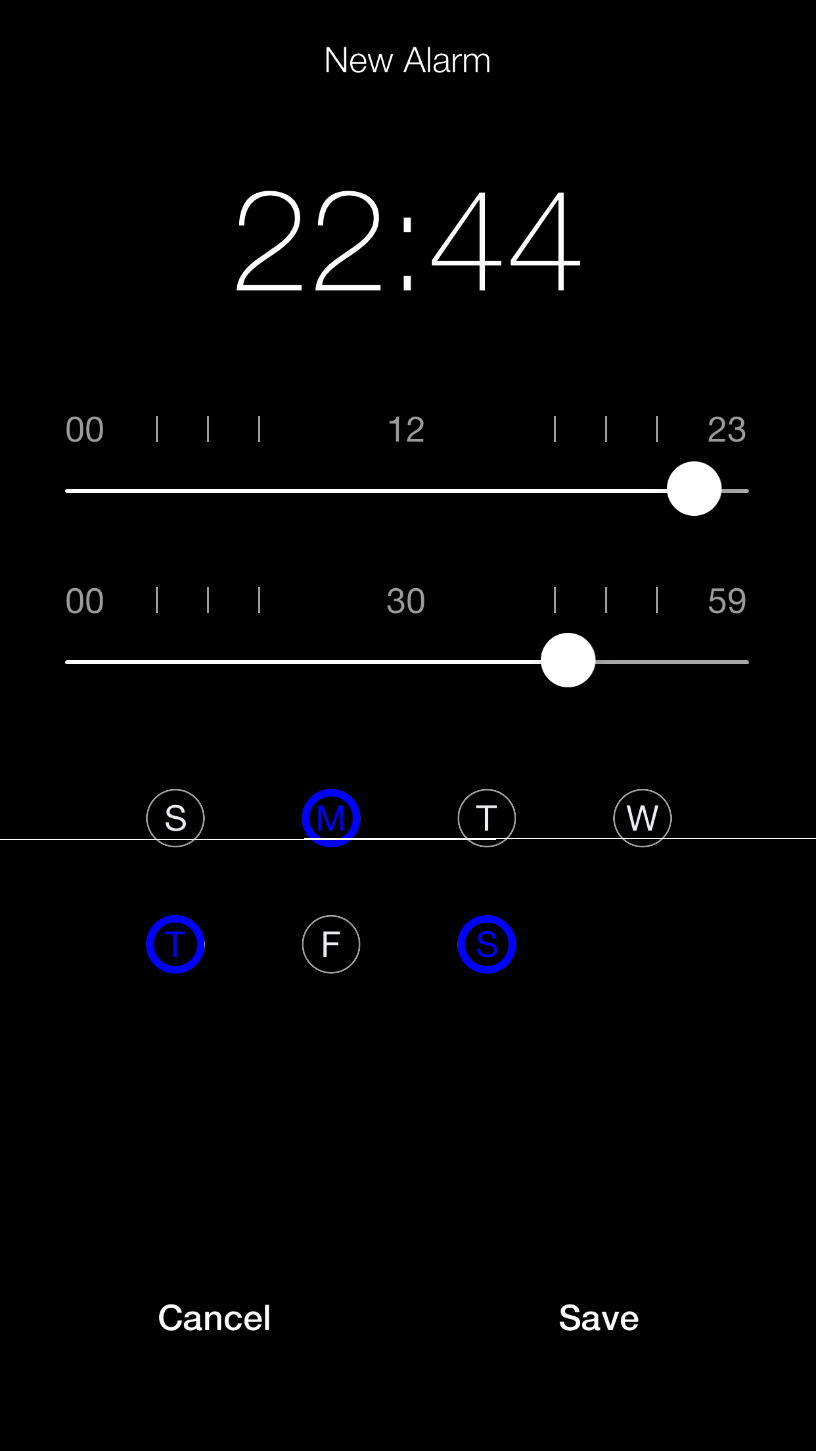The image displays a digital screen, likely from a non-iPhone smartphone, showing the interface for setting a new alarm. The background is entirely black, with the text "New Alarm" centered at the top in white font. 

Below this heading, in a larger white font, the time "22:44" is prominently displayed. Beneath the time, there are customizable sliders for setting the alarm. The first slider represents the hour, labeled with "00" on the left, "12" in the center, and "23" on the right, each separated by three lines. The slider tab is positioned slightly past "23" but not fully to the end. 

The second slider, for minutes, similarly has "00" on the left, "30" in the center, and "59" on the right, with three lines separating them. The tab on this slider is positioned just after the first line following "30".

Directly below the sliders are seven circles representing the days of the week: "S" for Sunday, a blue "M" for Monday, a white "T" for Tuesday, a white "W" for Wednesday, a blue "T" for Thursday, a white "F" for Friday, and a blue "S" for Saturday. A line runs horizontally through the days from "M" to "S".

At the very bottom of the screen, two spaced-out buttons are displayed: the first one labeled "Cancel" and the second one labeled "Save," both in white.

This detailed depiction captures the functional yet straightforward design of the alarm-setting interface.